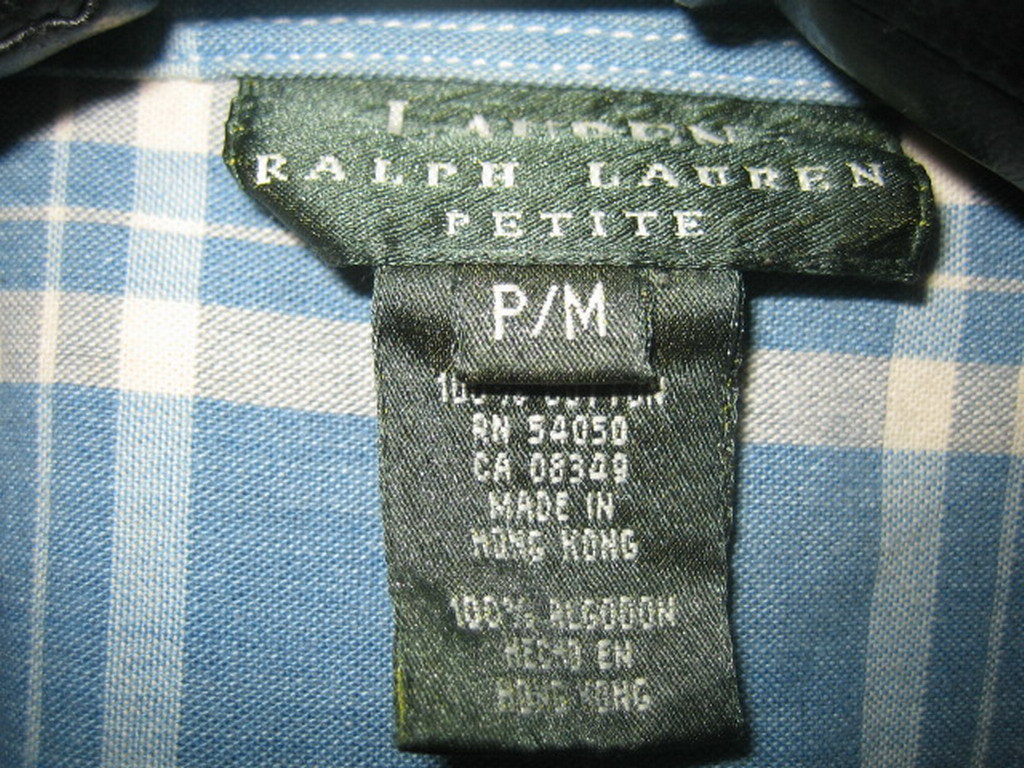The image showcases the interior of a Ralph Lauren jacket, with a glimpse of its black exterior. Dominating the view is the jacket's plaid lining, which seems to be composed of either pure cotton or a cotton blend. The layout of the lining strongly suggests the garment is indeed a jacket, reinforced by the presence of a visible tag. This tag, bordered in black material, prominently displays the brand name "Lauren Ralph Lauren" and indicates the garment's size as petite medium (P/M). Additionally, the tag specifies that the jacket is made of 100% Algodón (Spanish for cotton) and manufactured in Hong Kong. The tag also features a series of code numbers, further detailing its production origin.